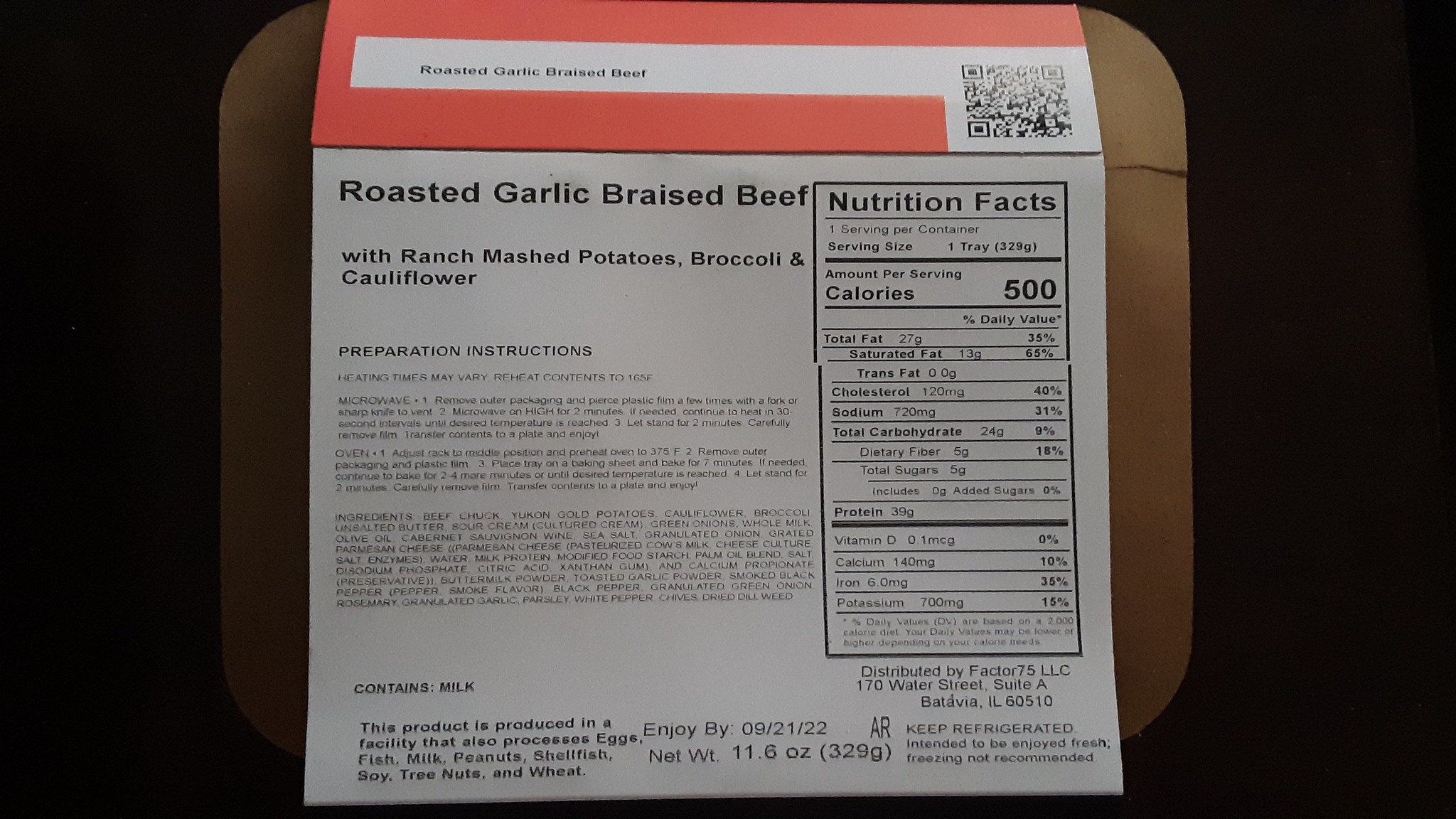The image features a white packaging label set against a black background. Centered on the label is a detailed description in black print. At the top left, the label reads "Roasted Garlic Braised Beef with Ranch, Smashed Potatoes, Broccoli, and Cauliflower." Below this, a section titled "Preparation Instructions" is followed by a block of text, although the print is too small to decipher. At the bottom of the label, it prominently states "Contains Milk," followed by a note that reads, "This product is produced in a facility that also processes eggs, fish, milk, peanuts, and shellfish."